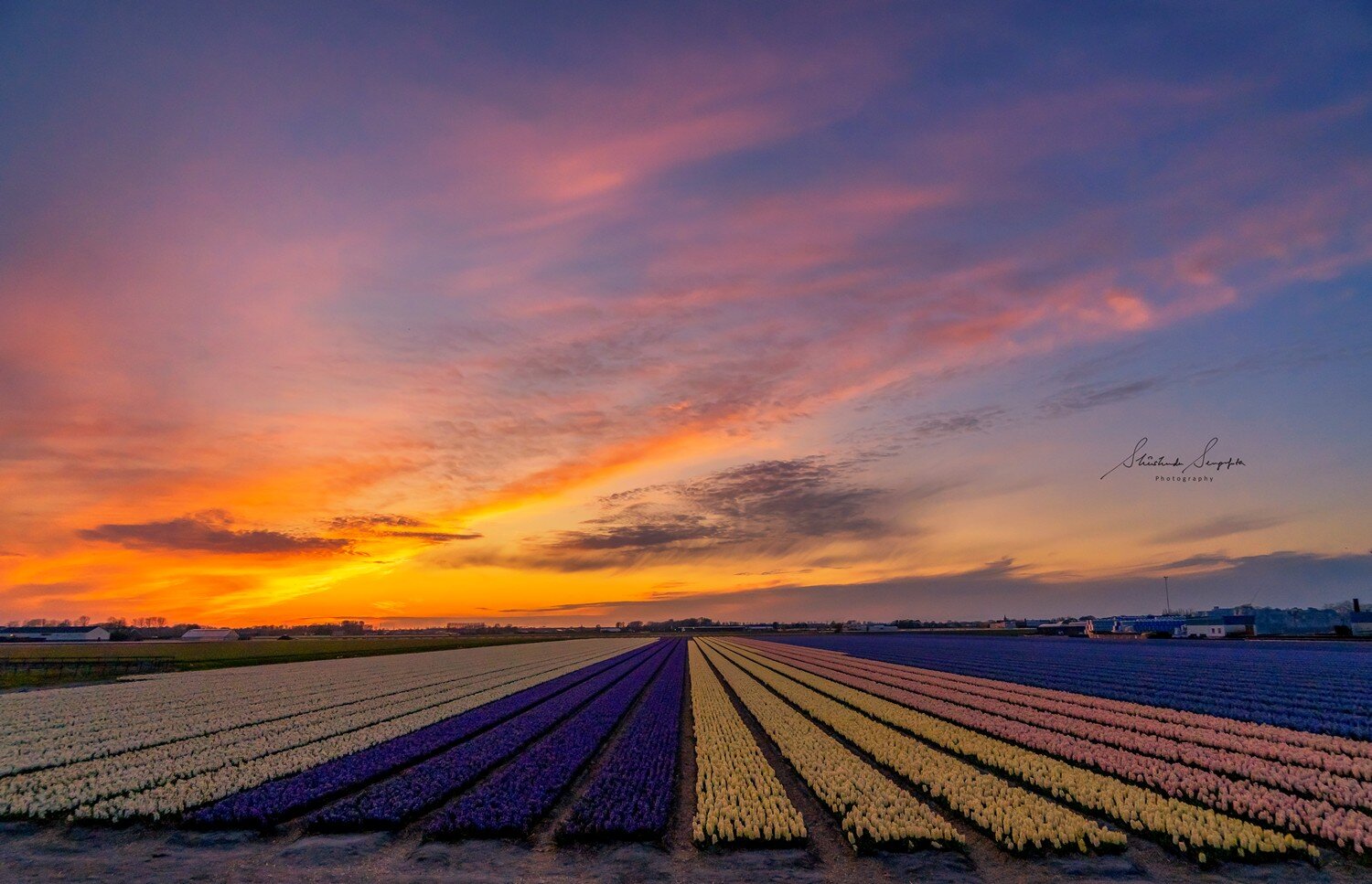A stunning photograph captures a panoramic view of a flower field at sunset. The horizon is positioned about three-quarters down the image, with the sky above adorned in an enchanting gradient of dark blue, mingling into pinks and fiery shades of orange and yellow. Clouds are scattered across the sky, with a hint of the setting sun peeking through the left side. Below the sky, a series of white barn buildings with roofs in various colors—black, blue, and one that appears to be transparent, possibly a greenhouse—stand prominently. Additional buildings and trailers edge the right side of the scene, accompanied by a tree line.

The foreground features a verdant clearing that transitions into meticulously arranged flower patches. Closest to the viewer, the rows begin with a mix of yellow and white flowers. These are followed by four rows each of deep purple, bright yellow, and then pink flowers. Further into the distance, the rows take on hues that seem to alternate between shades of purple and blue, extending far beyond the immediate view. The right side of the image includes the photographer's signature and the word "photography" in black, subtly marking the beauty captured in this landscape.